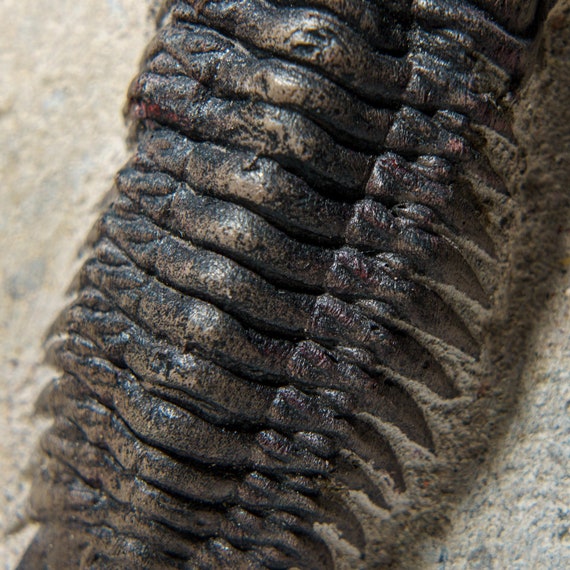This is a vertical, full-color close-up photograph of a small, heavily segmented creature with many legs, likely a pill bug, against a textured background. The background, which appears to be a mix of stone and sand with varying shades of grey and brown, suggests an outdoor setting. The creature itself has a dark brown to black coloration, with a brass-colored sheen in certain light. It exhibits numerous ridges running from its bottom to its top, resembling the underbelly of an ancient crustacean or trilobite, possibly a fossil from a prior era. On the visible left side, there are sharp, triangular wedges that resemble teeth-like structures. The intricate details of both the creature's segmented armor and the textured background create a striking contrast, highlighting the creature’s ancient and resilient form.